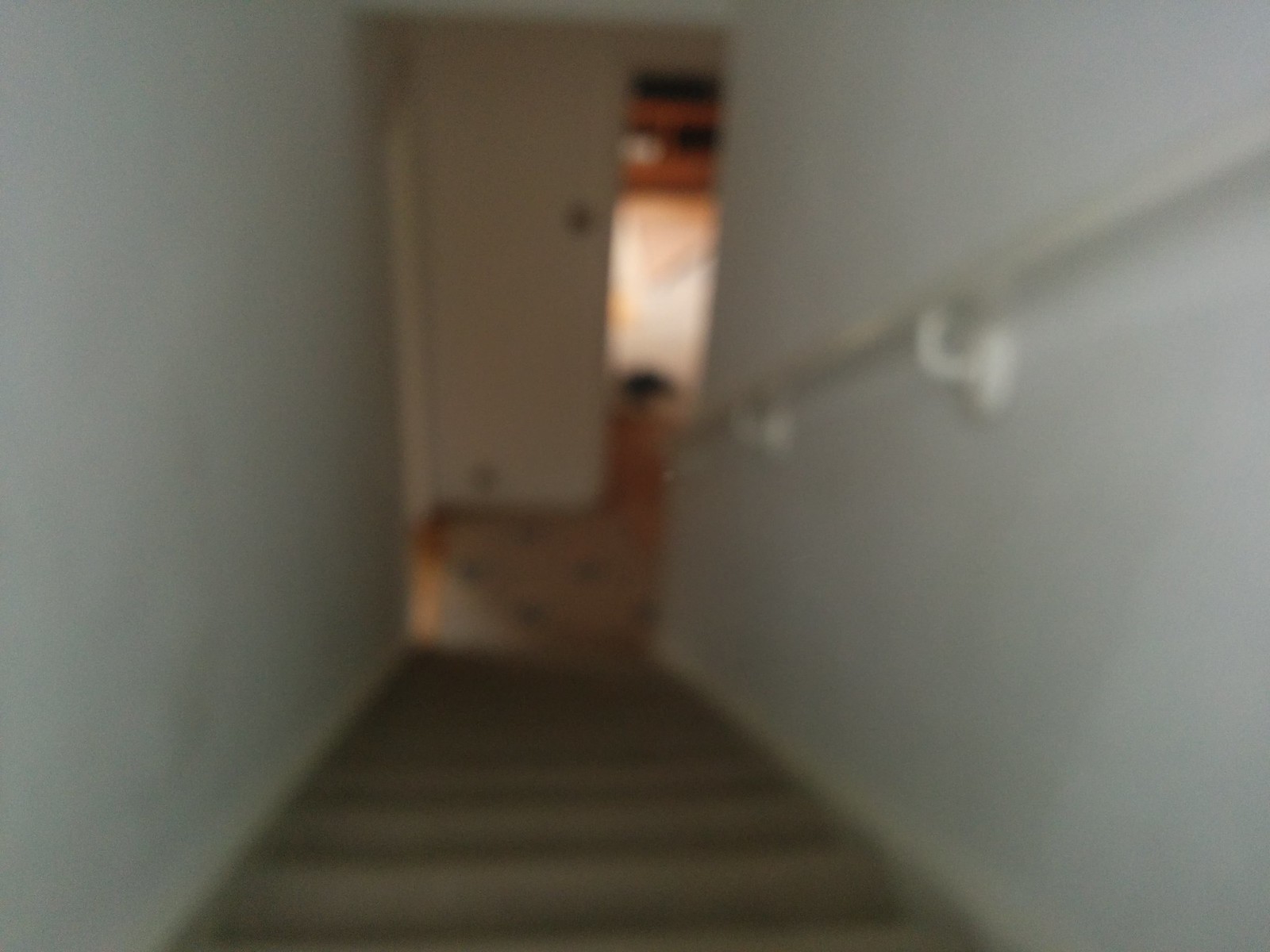The image depicts a very blurred photograph looking down a white-walled stairwell inside a house. The stairs are covered in tan carpeting, and a white handrail is affixed to the right wall with two white metal brackets. At the bottom of the staircase is an off-white or white rug, bordered by some decorations that are difficult to discern due to the blur. There is also a wall at the bottom, and to the right, possibly another stairwell or a room illuminated by natural light, suggesting the presence of a window. Additionally, there is a slightly open door on the left, hinting at more rooms or another level within the house. The overall setting is quite ambiguous due to the image's out-of-focus nature.